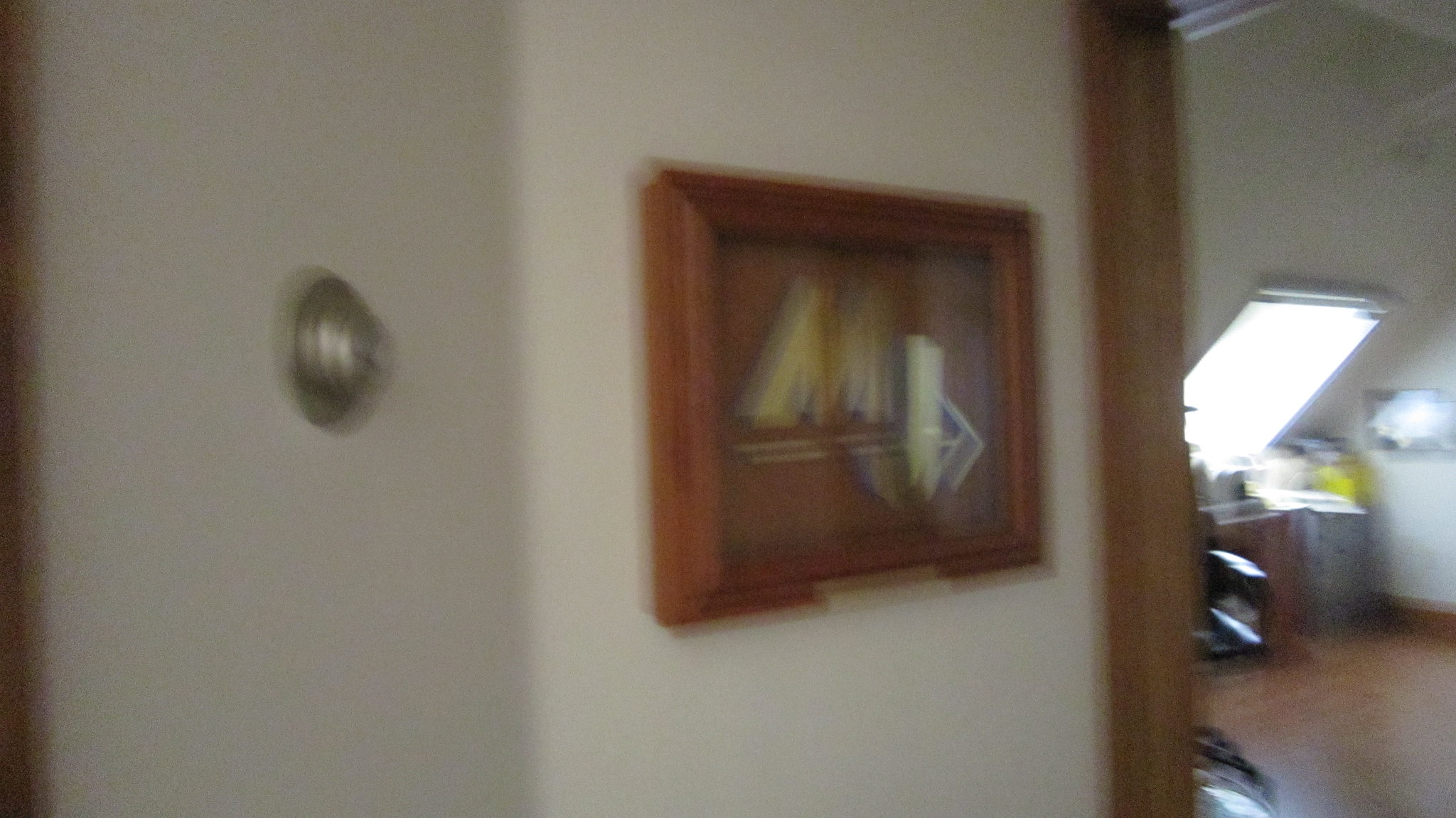The image depicts the interior of a building or house with predominantly white walls, though the overall quality appears blurry. On the left side of the image, there is a metallic circular object or perhaps a boat-like structure, though it's indistinct. Adjacent to this is a brown wooden picture frame, which houses an unclear image, but the presence of yellow and triangular shapes is noticeable. Further into the room, the light source seems to be a rectangular feature, possibly a window or a machine, though its exact nature is unclear. The room contains a mixture of colors including brown, white, green, and black, with a brown wooden floor completing the scene.